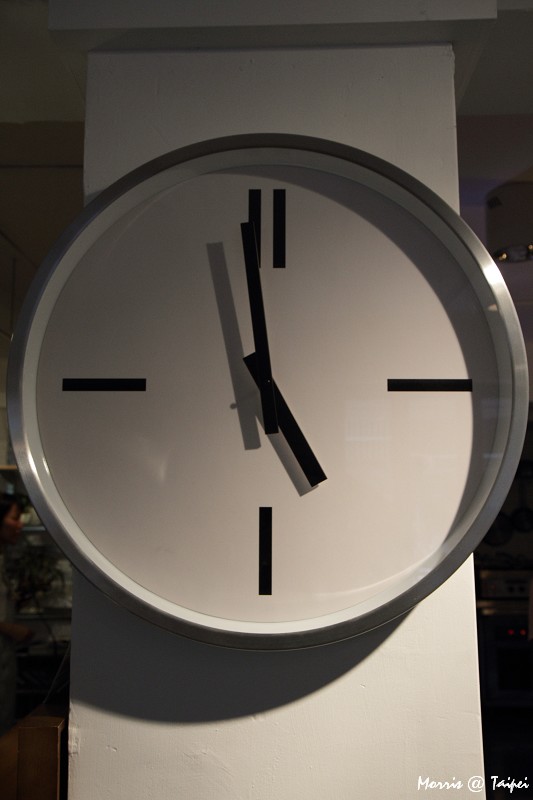In this image, a dark office interior serves as the backdrop, cluttered with papers and various office supplies. A wall adorned with a framed picture is contrasted by a light gray beam running vertically across it. Dominating the center of the wall is a prominent clock, featuring a sleek, silver metal casing. The clock's face is marked with minimalist black stripes, two for the 12 o'clock position and single stripes for the 3, 6, and 9 o'clock positions. Black hands indicate the time, casting a significant shadow due to the thickness of the clock's design.